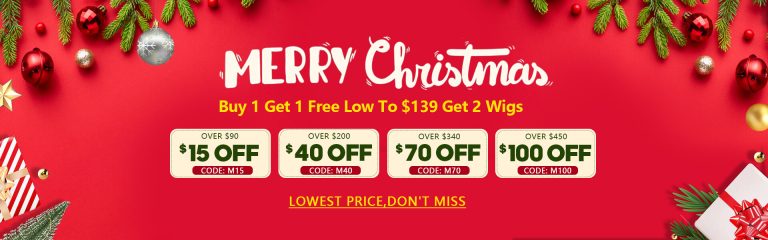This is a vibrant, color advertisement with a festive Christmas theme set against a white background. Each of the four corners of the advertisement features a rectangular area decorated with Christmas ornaments. The top left and right corners display red and silver ornament balls nestled in lush greenery from a Christmas tree. The bottom left and right corners, though mostly out of frame, show beautifully wrapped packages in red and white striped paper, adorned with red and white striped bows.

At the center of the advertisement, the text "MERRY CHRISTMAS" is prominently displayed. "MERRY" is written in bold, all-caps letters, while "Christmas" is elegantly scripted in cursive. Beneath this greeting, in bright yellow text, is a special promotional offer: "Buy One, Get One Free. Low to $139 dollars, get two wigs."

Below this offer, four white boxes are aligned side by side, each containing a different tiered discount. The first box reads, "Over $90, $15 off, code M15." The second box states, "Over $200, $40 off, code M40." The third box declares, "Over $340, $70 off, code M70." The fourth and final box announces, "Over $450, $100 off, code M100." Concluding the advertisement, an eye-catching yellow message at the bottom urges, "Lowest price, don't miss!"